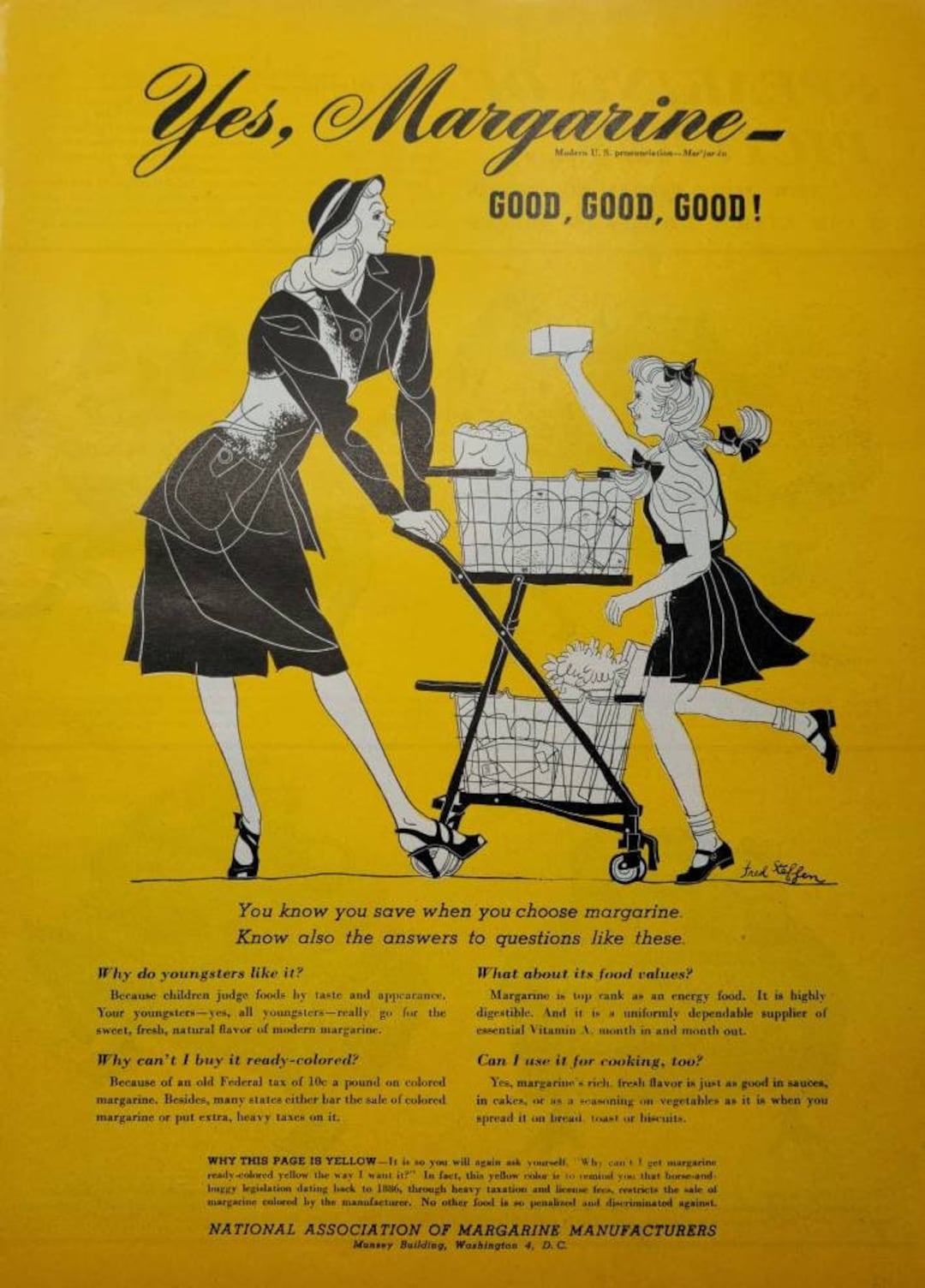This image is a vintage advertisement, likely from the 1940s or 1950s, featuring a detailed black and white illustration on a yellow background. At the top, in elegant cursive, the text reads, “Yes, margarine. Good, good, good!” The scene depicts a mother, dressed in a 1940s-style black business suit jacket, a skirt, and high heels, pushing a grocery cart brimming with groceries. She is accompanied by a young girl in a black apron dress with a white blouse, pigtails adorned with black bows, and black Mary Jane shoes with anklet socks. The child is eagerly holding up a box of margarine to her mother. Beneath the illustration, there are various black text details about margarine, addressing questions such as “Why do youngsters like it?”, “Why can’t I buy it ready colored?”, “What about food value?”, and “Can I use it for cooking too?” The advertisement concludes with the note that it is from the National Association of Margarine Manufacturers in Washington, D.C. The reason for uncolored margarine is explained as due to an old federal tax on colored margarine.